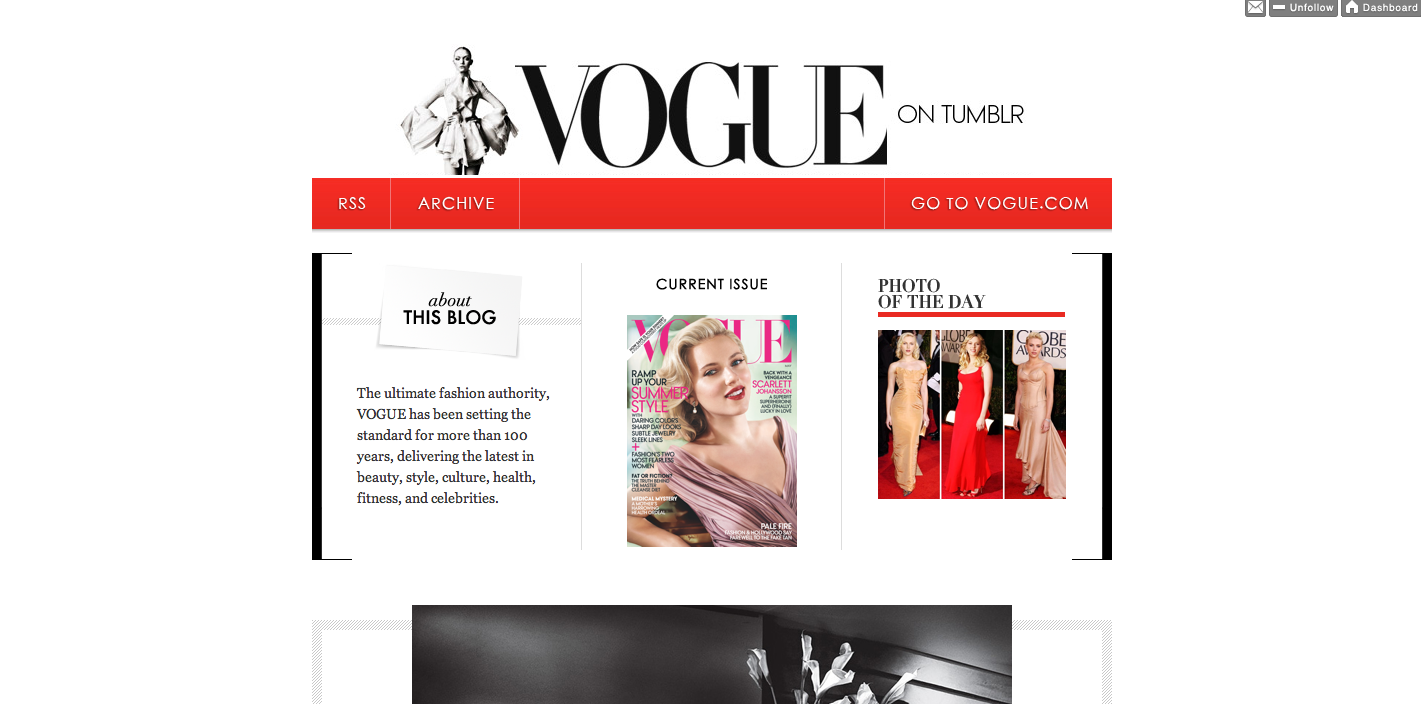Screenshot of Vogue's Tumblr Webpage:

The screenshot captures the Vogue website as viewed on Tumblr, showcasing the iconic Vogue logo prominently at the top. Below the logo, a stylish model is seen wearing a blouse characterized by fluttery sleeves. In the upper right corner, there are buttons for "Email," "Unfollow," and "Dashboard." Directly beneath the "Vogue on Tumblr" heading, a vivid red rectangular bar features white text buttons for "RSS" and "Archive."

On the right-hand side of the screen, the URL "gotovogue.com" is displayed next to a vibrant red button with white text. The webpage is segmented into three primary sections framed by large rectangular brackets. The first section, titled "About This Blog," describes Vogue as the ultimate fashion authority, setting standards for over a century by delivering the latest in beauty, style, culture, health, fitness, and celebrity news.

The second section highlights the current issue, featuring Scarlett Johansson in a retro-inspired dress with elements reminiscent of fashion from the 1920s to 1940s, emphasizing summer style. Below this, the "Photo of the Day" showcases three glamorous red carpet dresses from the Golden Globe Awards.

At the bottom of the screen, a partially cut-off black-and-white photograph is visible. The image appears to have an intricate geometric design, with a white twisted paper-like object and an indistinct background that might include a door or rectangular shapes, rendered in shades of gray and black.